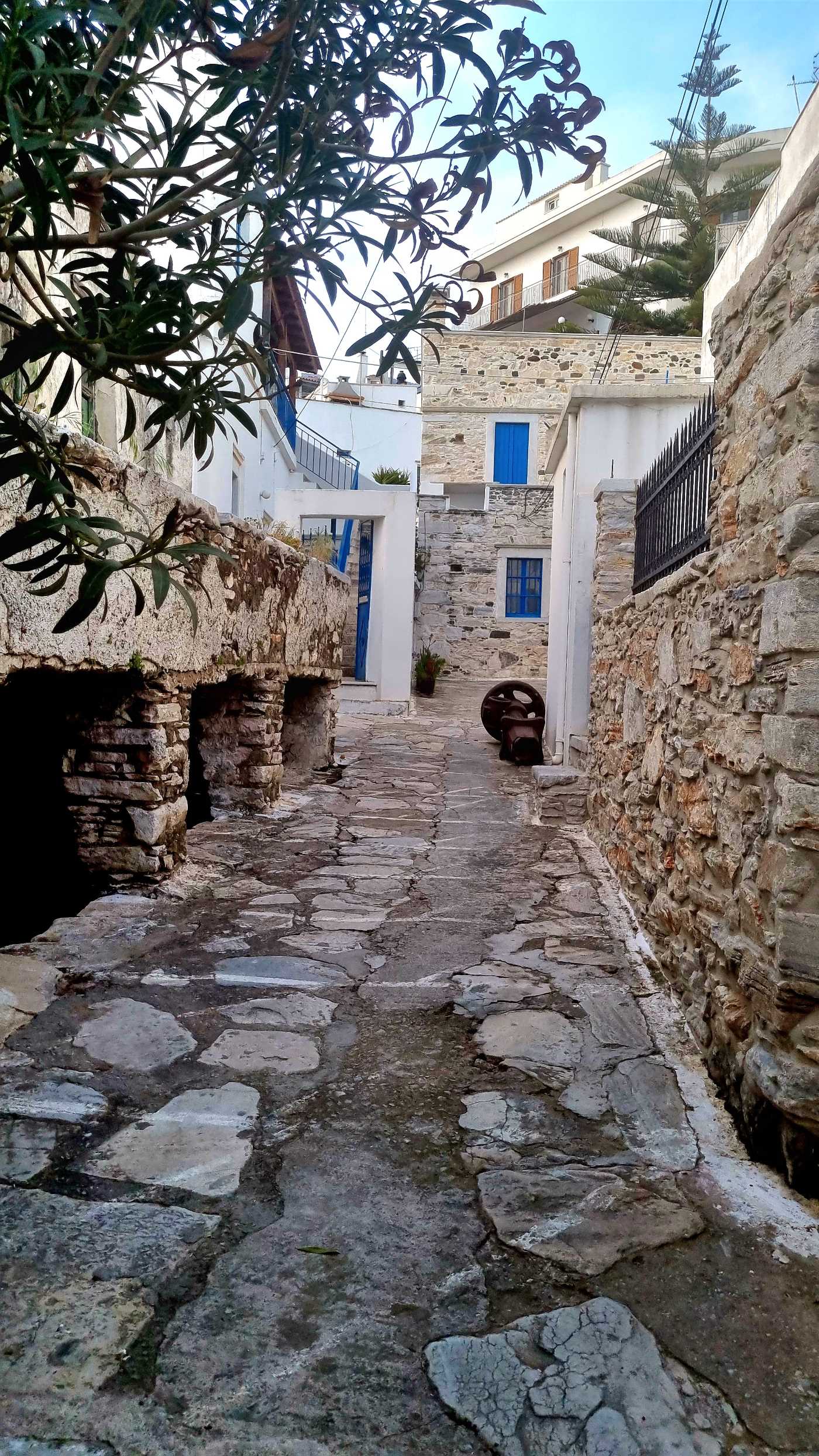The image depicts a picturesque outdoor alleyway with a cobblestone walkway made of white, gray, and brown stones, leading toward a series of rustic buildings. These buildings, constructed from a mix of tan, gray, black, and white rocks, are multi-storied and exhibit blue windows, a blue door, and a blue staircase visible on the left-hand side of the distant structure. Some sections of the buildings feature white portions and wooden archways. Overhead, green tree branches with dark green leaves hang into the frame, while telephone wires crisscross the blue sky above. The scene evokes a quaint, historical ambiance with its carefully detailed stonework and charming architectural elements.